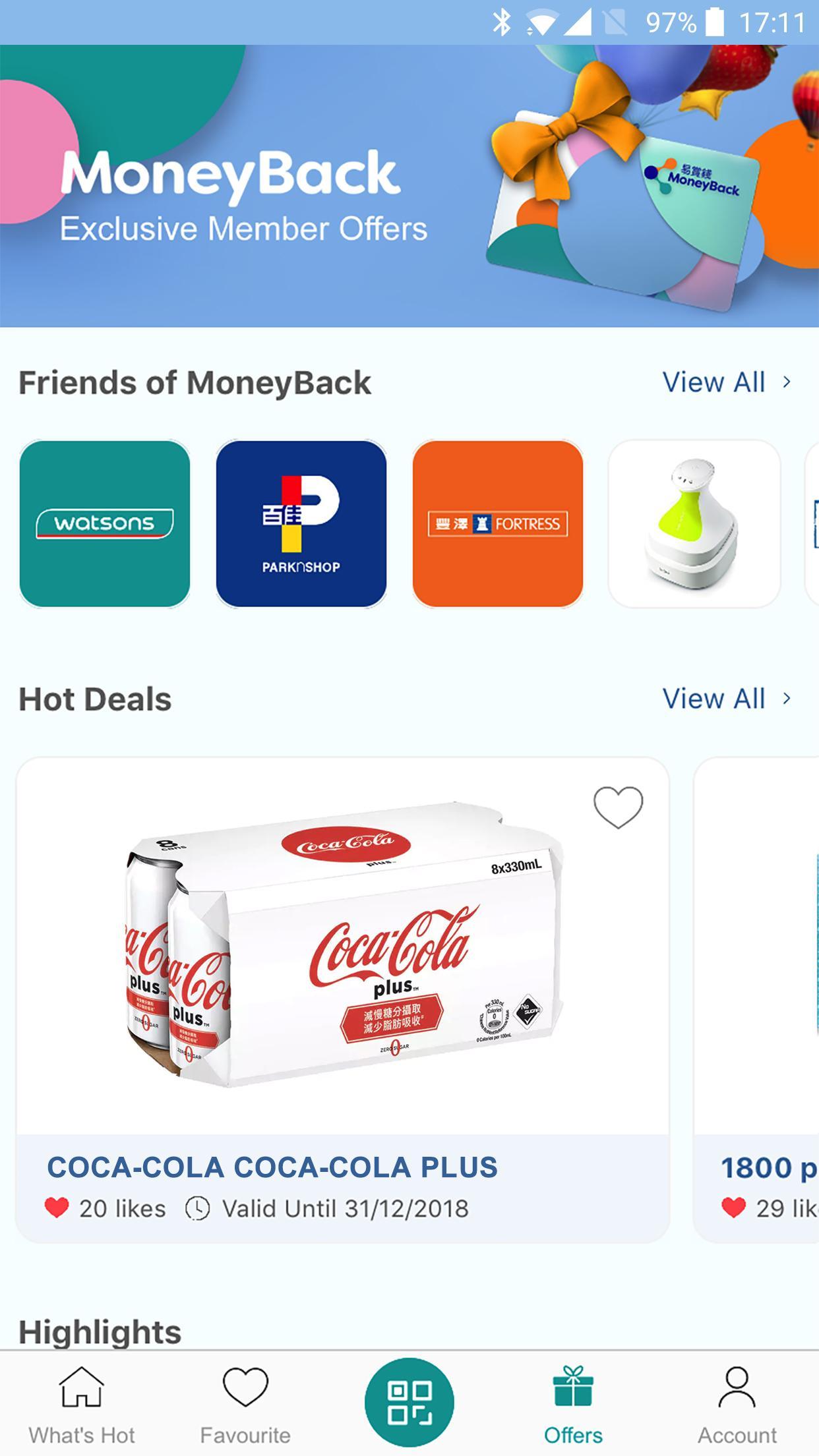Screenshot Description of the Money Back App Interface:

The screenshot is in portrait mode, featuring the interface of the Money Back app. 

- **Top Section:**
    - **Status Bar:** A light blue stripe runs across the top. On the upper right, the battery shows 97%, and the time is 17:11.

- **Main Content:**
    - **Background:** The app is displayed in landscape mode.
    - **Left Side:**
        - A pink half-circle and part of a green circle are visible, adding a colorful element to the design.
    - **Right Side:**
        - A graphic of what appears to be a gift card with a gold bow is present. Several balloons and a strawberry icon are also part of the visual.
        - **Text:** "Money Back Exclusive Member Offers".
    - **Next Row:**
        - **Text:** "Friends of Money Back."
        - **Right Side:** A live button labeled "View All".
    - **Grid Section:**
        - Four square icons are displayed, representing different stores or services: Watson's, Park N Shop, Fortress, and an unidentified icon.
    - **Next Row:**
        - **Text:** "Hot Deals."
        - **Right Side:** A live link labeled "View All".
    - **Highlighted Deal:**
        - **Image:** Coca-Cola Plus bottle with a lot of Asian writing on it.
        - **Icons:** A heart icon to favorite, showing "Coca-Cola Plus". It has 20 likes.
        - **Validity:** "Valid until 31/12/2018".
    - **Adjacent Deal:**
        - A partial image of another product that would require scrolling to view fully.
        - **Text:** "1800P" with 29 likes.
    - **Footer Section:**
        - **Text:** "Highlights", "What's Hot", "Favorites".
        - Four main icons:
            - **Green Circle:** Contains what appear to be various icons.
            - **Offers:** Labeled in green.
            - **Account:** Indicates user account settings or information.

This screenshot provides an overview of the Money Back app interface, showcasing member offers, store icons, promotional deals, and relevant user interface elements.